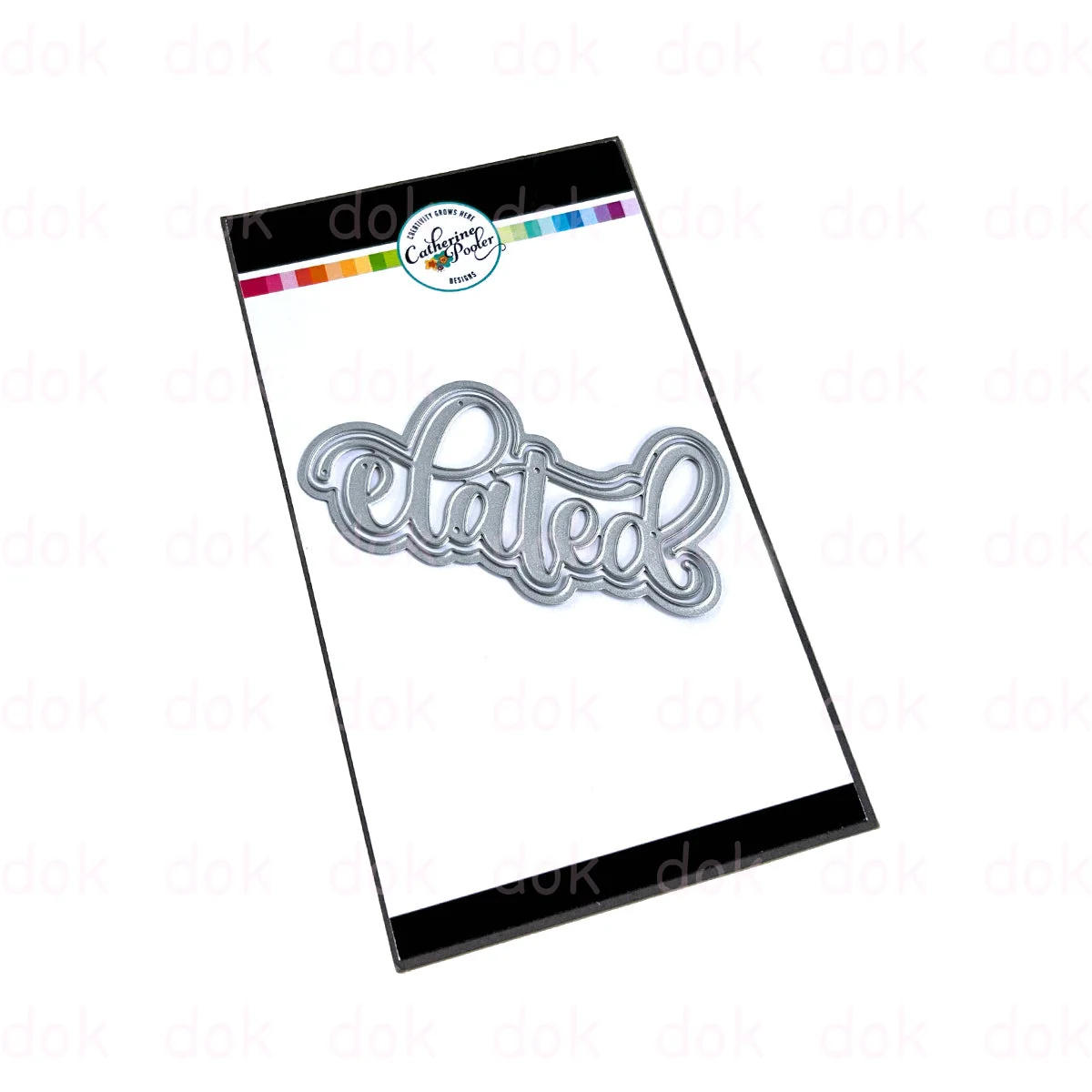The image showcases a rectangular drawing pad or tablet that resembles a digital scratch pad. At the top of the device, there's a color palette featuring a gradient starting from red and progressing through orange, yellow, green, blue, and purple. In the middle of the pad, there's a prominent cursive word "Elated," rendered in a metallic silver color that creates a 3D effect, as if drawn by a 3D pen. This word is outlined in silver as well and sits on a white screen. Overlaid faintly across the white background are the letters "DOK" in gray, serving as subtle watermarks. Additionally, there appears to be a label near the top, possibly a sticker, with the words "Catherine Pooler" on it. The overall design closely mimics that of a laminated card or a digital screen, slightly angled to resemble the size of a cell phone.